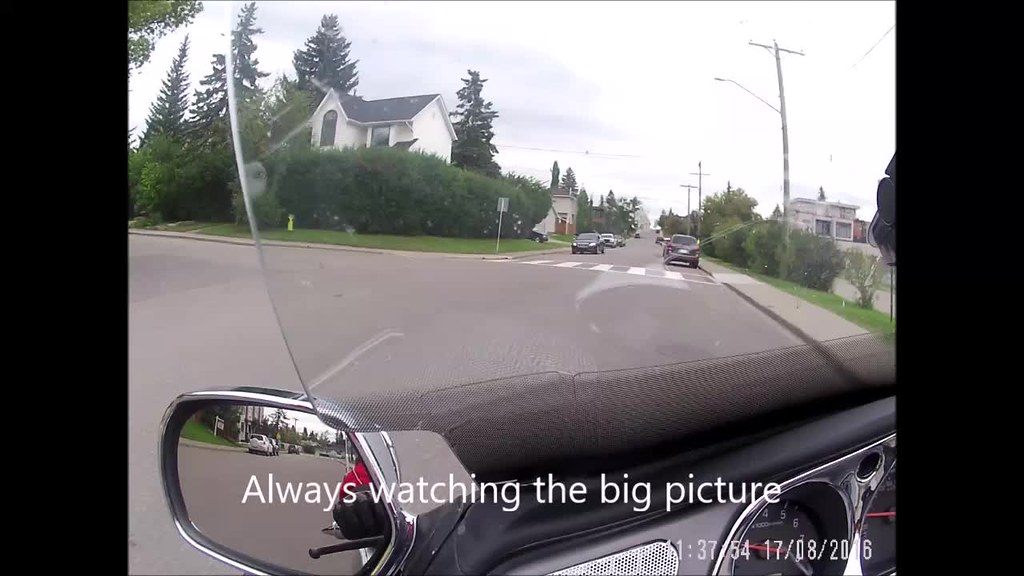The image captures a dynamic view from the perspective of a motorcyclist. The scene is framed by a rounded windshield, flanked by a chrome wing mirror and the edge of a speaker. In the foreground, the black-and-chrome dials of the speedometer are prominently visible. Reflected in the wing mirror, the motorcyclist's black-gloved hand and red-arm sleeve grip the handlebars, with the brake lever immediately in front.

The backdrop reveals a suburban intersection in the United States, marked by distinct architecture. Dominating the street corner is a two-story house with two prominent gable ends, surrounded by large bushes and evergreen trees. Adjacent to the house is a green fire hydrant. The view up the hill indicates a steep gradient, with cars parked on both sides of the road and a zebra crossing cutting across the junction.

Electrical poles and lampposts line the pavements, accompanied by neatly trimmed bushes. The road is flanked by additional houses on either side, adding to the picturesque suburban setting. Superimposed on the photograph, the words “Always watching the big picture” are displayed in white font at the bottom. Additionally, a timestamp and date, “11:37:54” and “17.08.2016” respectively, are printed on the bottom right corner.